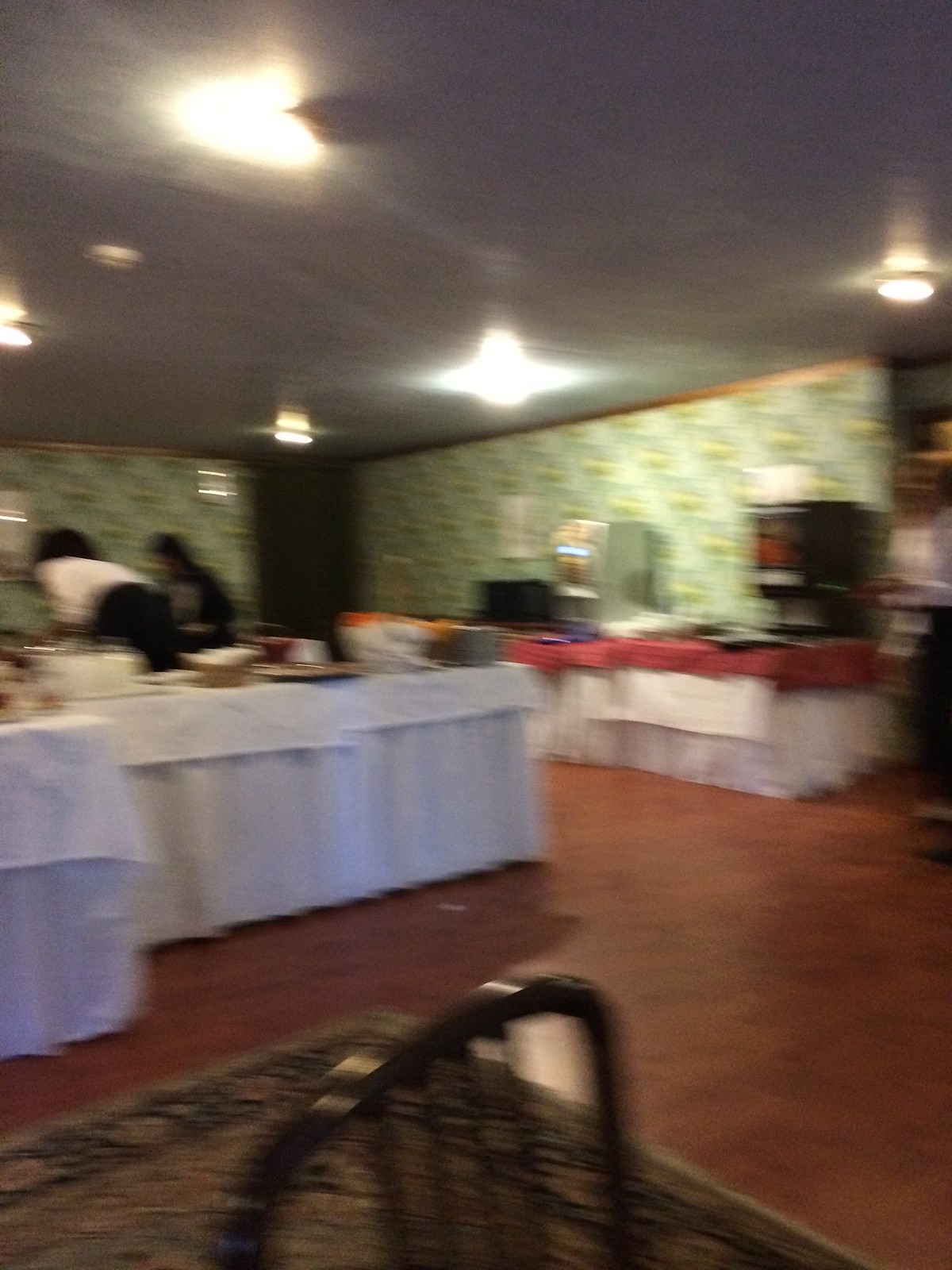This image, taken indoors, is very blurry and out of focus, making it difficult to see fine details clearly. The scene appears to be a restaurant or banquet hall with a dimly lit ceiling featuring about half a dozen lights. The walls are adorned with green and white wallpaper that includes gold patterns. In the center of the image, there's a doorway flanked by walls to the left and right.

The room contains two tables with white tablecloths, one of which also has a red tablecloth over it. These tables appear to hold various serving devices, such as drink dispensers, plates, and bowls. Two barely visible people are bending over near a table on the far left side of the photograph.

The floor is made of reddish dark hardwood, with a large rug partially visible in the foreground. Additionally, the back of a dark-colored chair with a metal frame is closest to the camera, giving a sense of depth to the image.